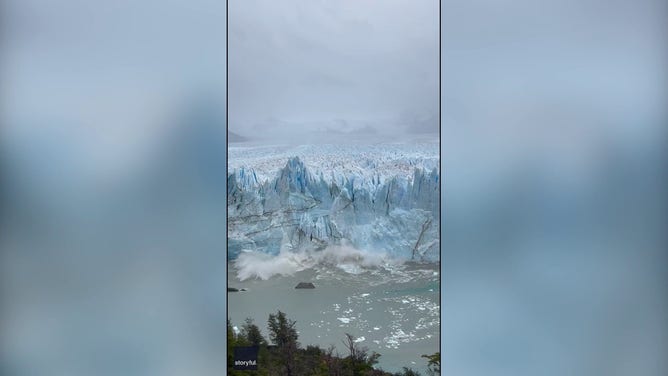The image, captured on an iPhone, is a striking vertical composition divided into three segments. The central section showcases a colossal light blue iceberg crumbling into a grayish body of water, with white, foamy waves erupting from the impact. The glacier itself stretches infinitely into the distance, accented by jagged peaks and distinct, layered fault lines filled with dirt. In the background, snow-covered mountain ranges mingle with a gray, cloudy sky, adding to the icy aesthetic. A sliver of green hills and trees is visible beneath the glacier, providing a touch of color to the stark, frozen landscape. The left and right segments of the image are blurred rectangles, perhaps highlighting key parts of the iceberg or water, creating a dramatic and surreal triptych effect. The word "Storyful" is placed at the bottom, anchoring the vivid scene.